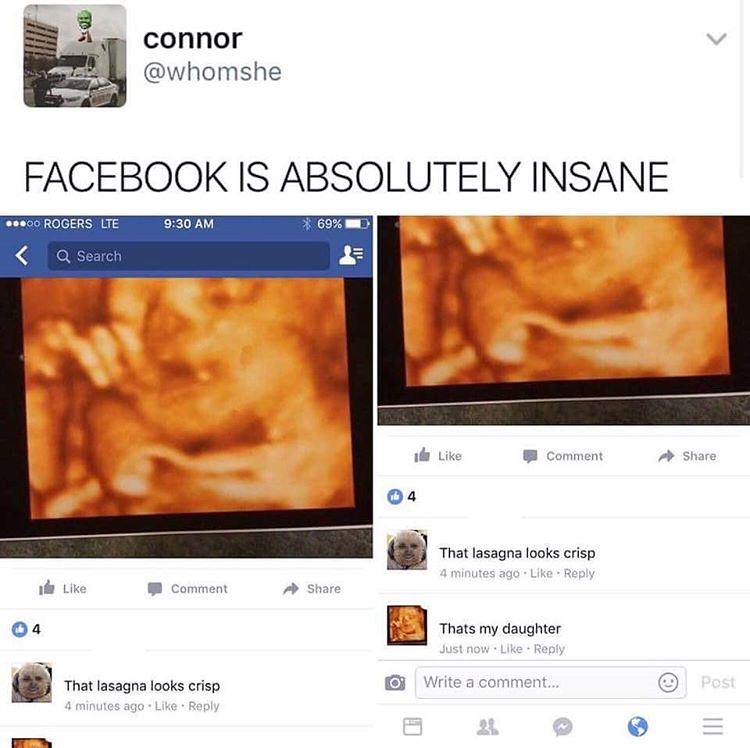This image is a screenshot of what appears to be a post on Instagram, featuring a Facebook post by a user named Connor (@WHOMSHE). The post's header includes a logo at the top left corner showing a profile picture of a large green-headed man standing on a white truck with a police car in front of it. Below Connor's name, the caption reads in bold capital letters: "FACEBOOK IS ABSOLUTELY INSANE." The post showcases two close-up photos, side by side, that initially seem to be pieces of lasagna. However, upon closer inspection, these images are actually detailed ultrasound images of a baby, with the baby's hand visible in front of its face. At the bottom of the post, there are comments from two users: one named "that lasagna looks crisp," featuring an icon of a man, and another named "that's my daughter," with a close-up of a baby's face as their profile picture. The bottom portion of the screenshot includes the usual Facebook layout elements, such as the "write a comment" section and various icons, along with indications of recent activity.